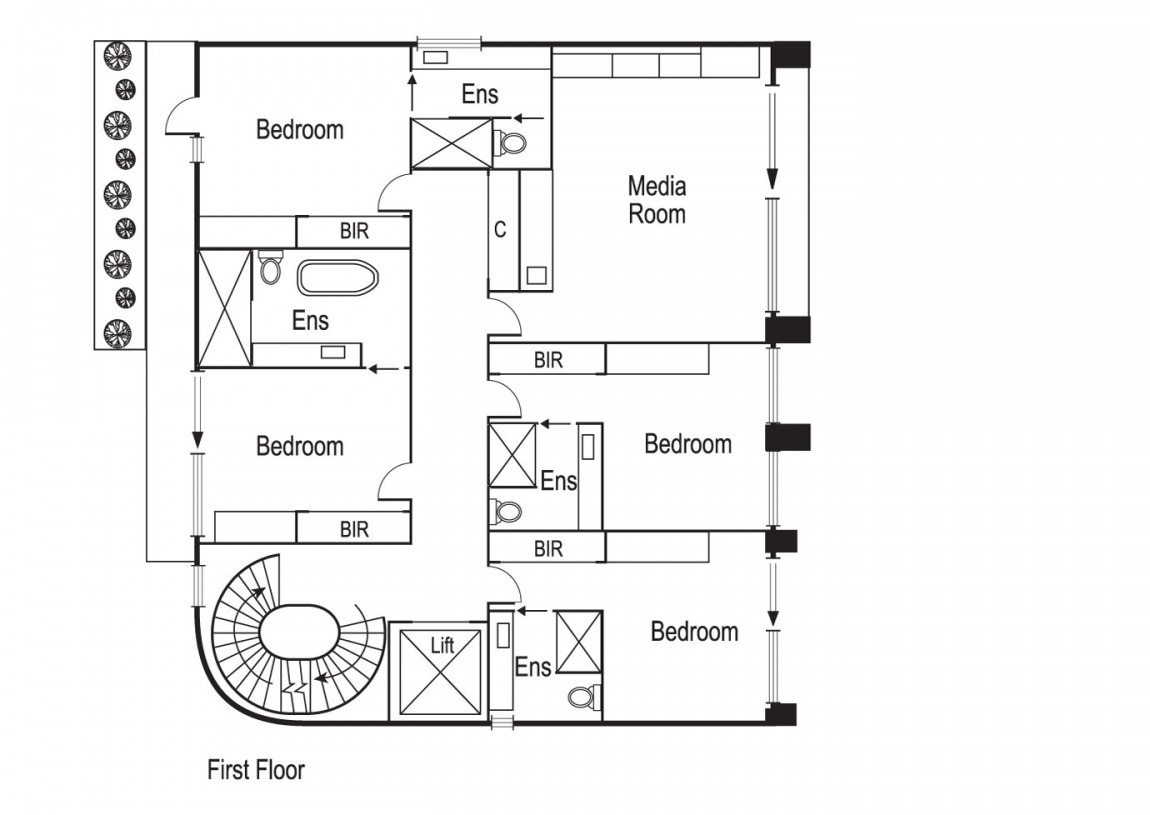This black-and-white diagram presents detailed blueprints for a new-build home, with a nearly square overall shape. The focus is on the first floor layout. A stairway is visible, leading to the second floor. The first floor features an elevator positioned centrally. Adjacent to the elevator is a small bathroom that connects to a bedroom. Proceeding down the hallway, another bedroom is located on the left side, with an attached bathroom. Further down the hallway, another bedroom can be found, featuring an access point to a porch. On the right side of the hallway lies a spacious media room, the largest room on the first floor. There is also an additional bedroom on this floor. In total, the first floor comprises four bedrooms, each paired with its own bathroom, ensuring ample convenience and privacy for its occupants.